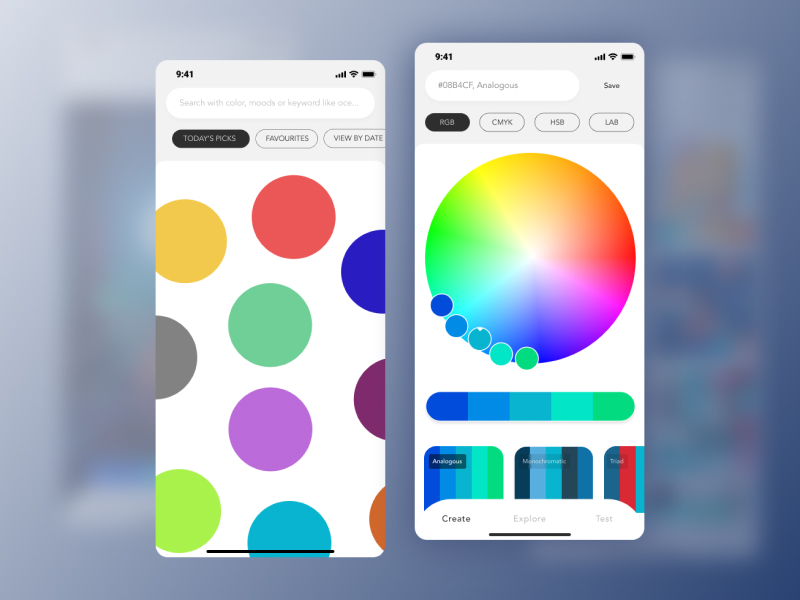The image displays two smartphone screens, each showcasing the same interface for a color management tool. The primary phone in the foreground is clearly visible, while the background features blurred phones to maintain focus on the main subject. Both phones show a time of 9:41 and have full Wi-Fi signal strength and battery life.

The main screen highlighted is organized with several distinct elements:

- **Color Moods and Keywords Search**: At the top, there is a search bar labeled "Color Moods and Keywords," accompanied by colorful polka dots in hues such as yellow, red, blue, gray, green, purple, dark purple, lime green, navy blue, and part of an orange.
- **Button Status**: A prominently black button labeled "Today's Pics" in white text is selected, alongside two additional options: a circle button for "Favorites" and another for "View by Date."
- **Advanced Settings**: Another phone at the same time, 9:41, mirrors the settings of the first device. It features a hashtag descriptor "8b 4c f analogs RGB," with its black button selected and showing white text. Options for "CMYK," "HSB," and "Lab" are also displayed.
- **Color Wheel and Shading Options**: Below these settings, there is a vibrant color wheel with gradients ranging from lime green to dark blue. Adjacent to it is a shading slider depicting a gradient from dark blue to light blue, then transitioning to lime green.
- **Navigation and Actions**: At the bottom of the screen, the word "Explorer" is underlined, flanked by a "Create" button to the left and a "Test" button to the right.

The overall functionality displayed allows users to manage and explore the red, blue, and green aspects of their phone's color settings in a detailed and comprehensive manner.

This caption provides a thorough description of the smartphone interface, detailing each element for clear understanding.